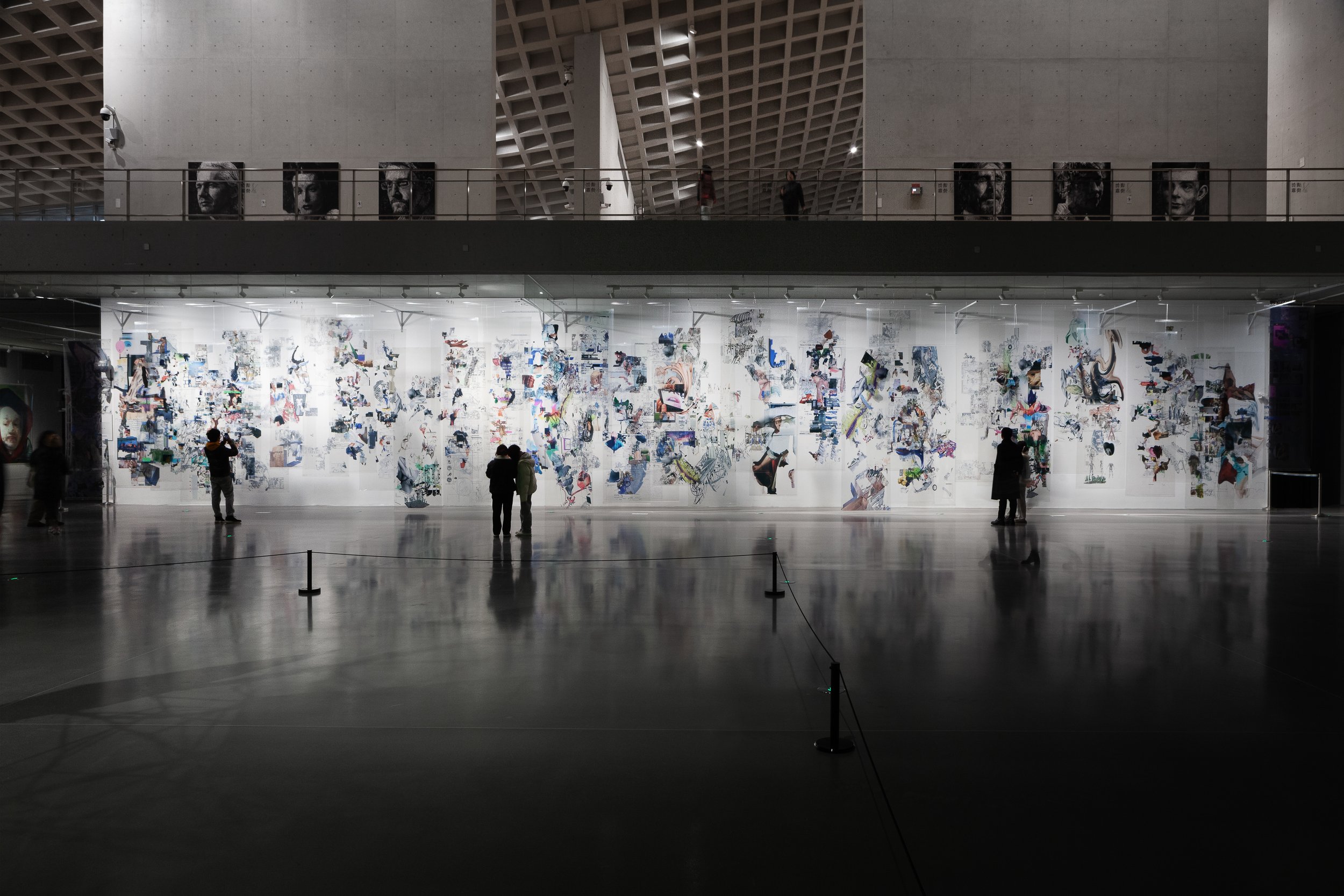The image depicts the interior of an art gallery with a modern aesthetic. The foreground features a large, shiny gray floor, partially enclosed by a rope barrier in the bottom left corner. The focal point is a big white wall adorned with vibrant pop art, showcasing a variety of colorful designs and drawings that are hard to discern clearly but captivate the onlookers. Approximately five people stand in front of the wall, some examining the art while others take photographs of it. The room itself is dimly lit, with spotlights illuminating the artwork, creating a striking contrast against the dark surroundings. Above this main exhibition area, there is a second-floor balcony with a gray rectangular floor, which has a railing adorned with six black-and-white photographs of people's faces. The ceiling extends upwards, featuring a distinctive waffle pattern composed of recessed squares, adding to the architectural intrigue of the space.